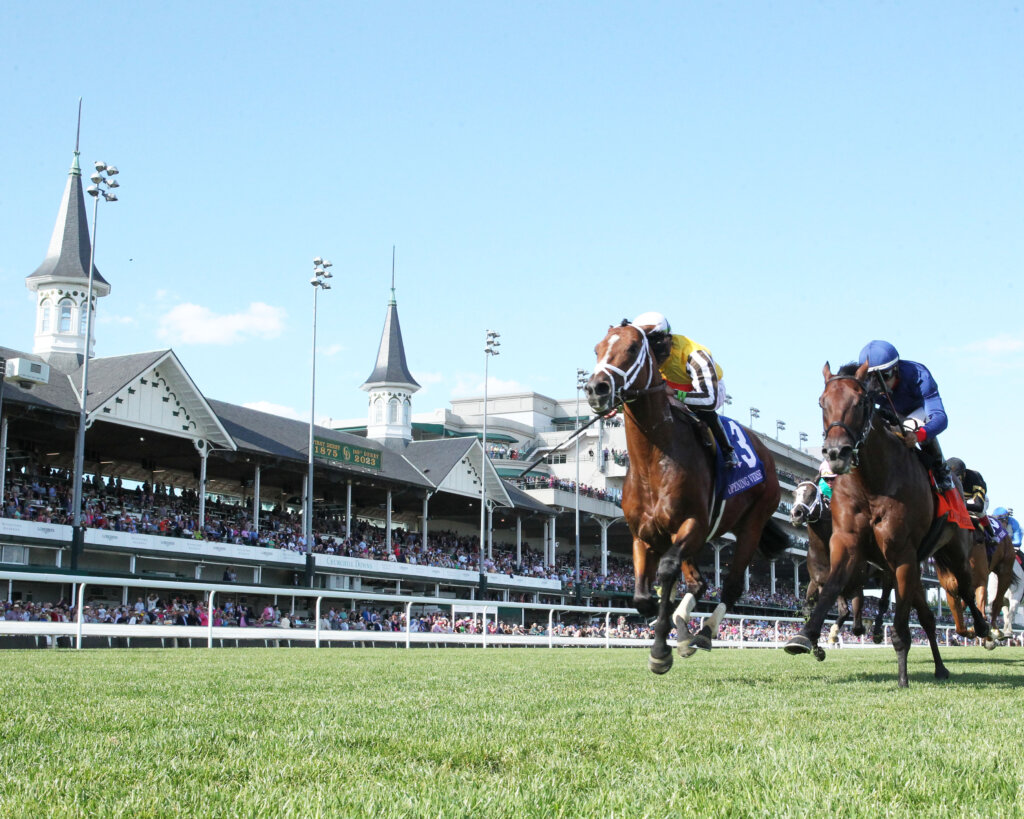This is a detailed photograph of a horse race taking place on a lush, green turf. The image is captured from a low, ground-level perspective, giving a dynamic view of the racing action. Two brown horses dominate the foreground, both in mid-stride, with their jockeys leaning forward intensely. The horse slightly ahead has a white blaze on its nose and is ridden by a jockey wearing a yellow shirt with black and white striped sleeves. The horse next to it is solid brown, ridden by a jockey in a blue shirt and helmet. Both horses are racing towards the left side of the image, neck and neck.

The backdrop features a grand, sprawling stadium that stretches across the entire width of the photo. The stadium, adorned with multiple, sharply pointed steeples or towers, is filled with hundreds of spectators clad in a multitude of colors. The seating is packed from the ground level up to the second tier, highlighting the event's popularity. A white fence separates the racetrack from the stands, and large lights are spaced evenly along the structure, likely for evening races. The sky above is a light blue with a few small clouds scattered on the left, adding to the picturesque quality of the scene. The energy and excitement of this high-stakes race are palpable, capturing a moment of intense competition in a beautiful, classic racetrack setting.